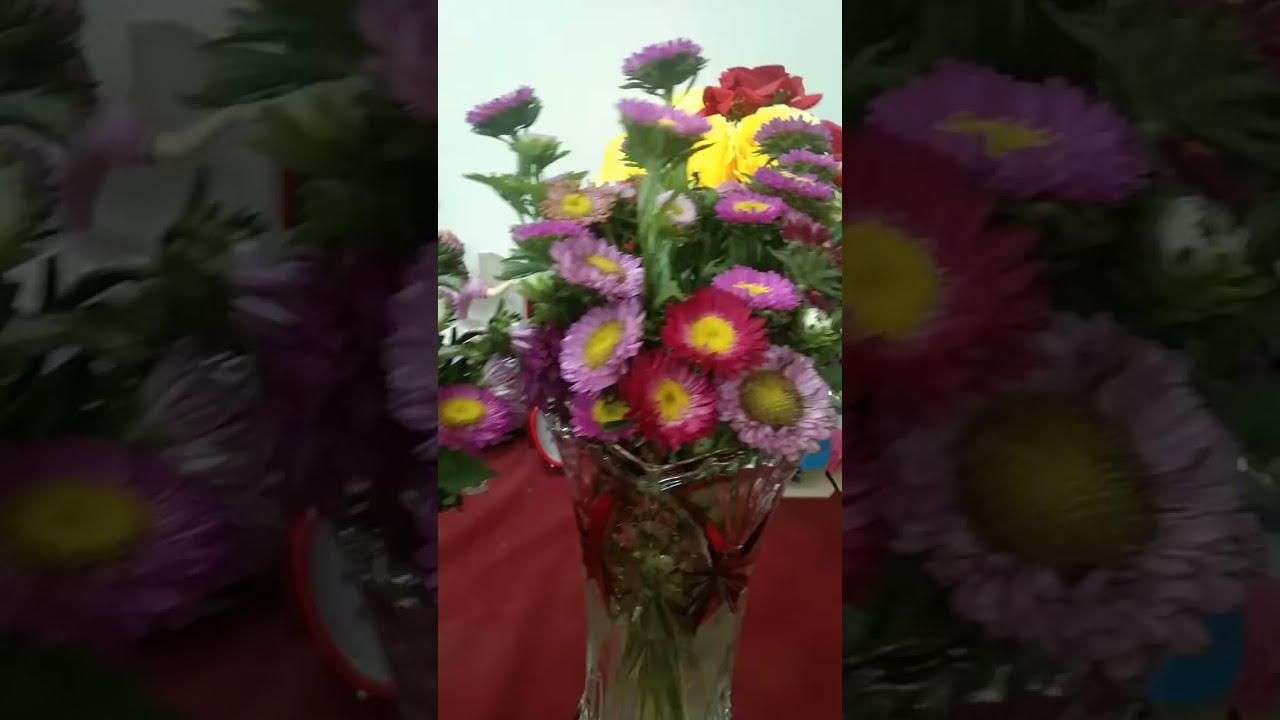In this image, a clear crystal vase filled with a vibrant bouquet of flowers is prominently centered on a red tablecloth. The vase holds an array of colorful daisies, predominantly in bright pink, lavender, and hues in between. Each daisy features short, slender petals and yellow centers, with delicate, fine elliptical green leaves adorning the stems. In the background, you can glimpse hints of yellow and red roses, suggesting another vase nearby, though it remains out of view. The backdrop appears to be a light blue wall, adding a serene contrast to the lively floral arrangement. The photograph is framed by enlarged and darkened images of the pink daisies, creating a border effect. Subtle, indistinct items, possibly including a red alarm clock, are visible in the background but remain unclear. The overall composition hints at a screenshot from a mobile device, possibly captured from an app like TikTok or Instagram.